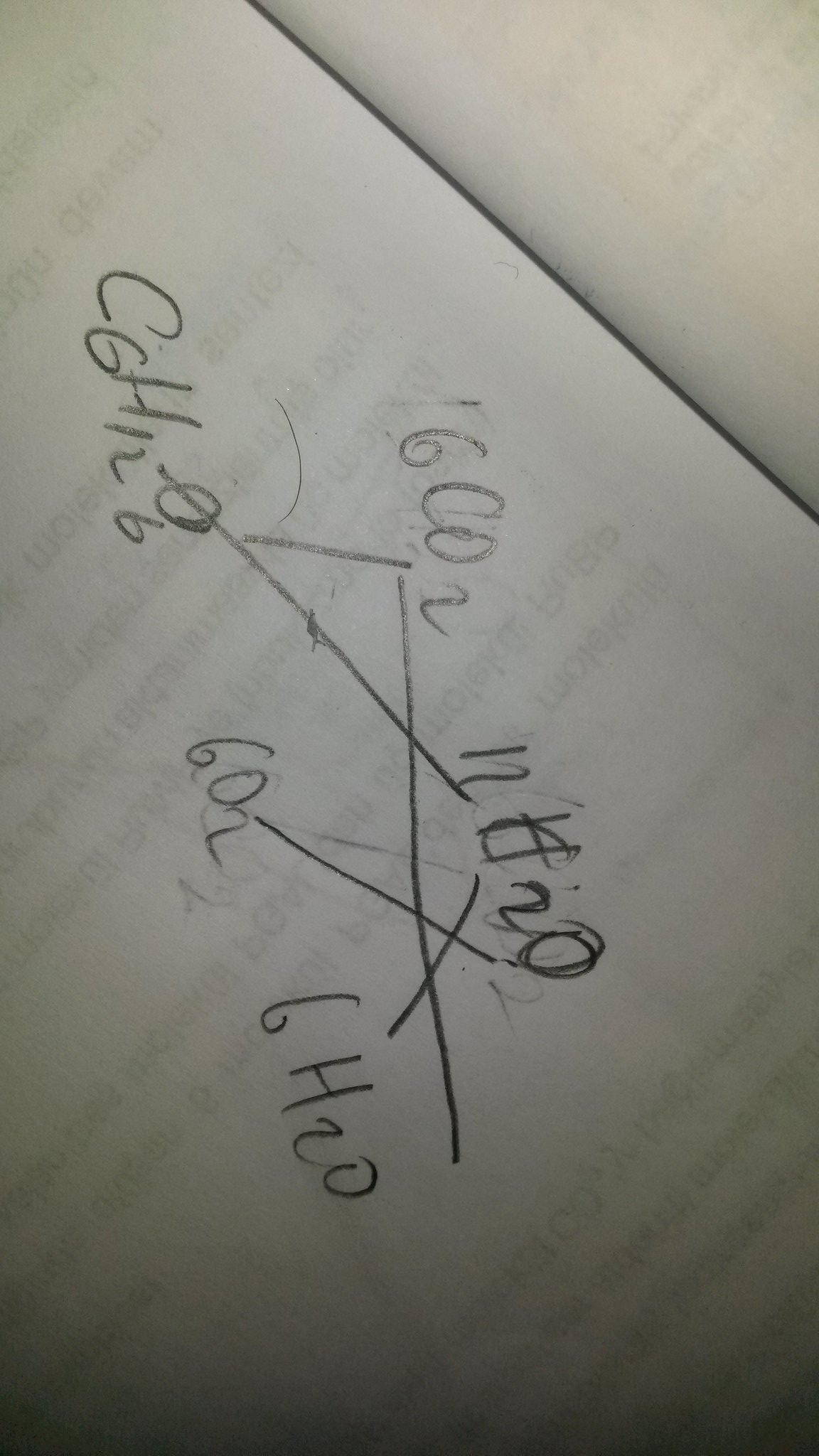This appears to be an image of a handwritten chemistry problem involving a complex chemical equation, with the paper oriented sideways. The core illustration consists of a geometric shape where a mix of lines and angles suggests spatial relationships between chemical compounds. A central diagonal line intersects the shape, forming a triangle - one angle of which is 40 degrees and another at 90 degrees.

At the apex of this triangle is the chemical formula \(16CO_2\). On the right side of the diagram lies \(NE, possibly NH_2O\). Down to the left corner, the formula \(CGH_2O_6\) is written, with \(6O_2\) and \(6H_2O\) positioned towards the right.

These chemical notations are connected by various intersecting lines, including a significant cross-line that ties \(NH_2O\) with \(6O_2\) and \(6H_2O\) below it. Another critical diagonal line links \(CGH_2O_6\) with \(NH_2O\), emphasizing the relational structure of the equation components. Despite the intricate design, the problem's solvability and context remain unclear due to the observer's limited expertise in chemistry.